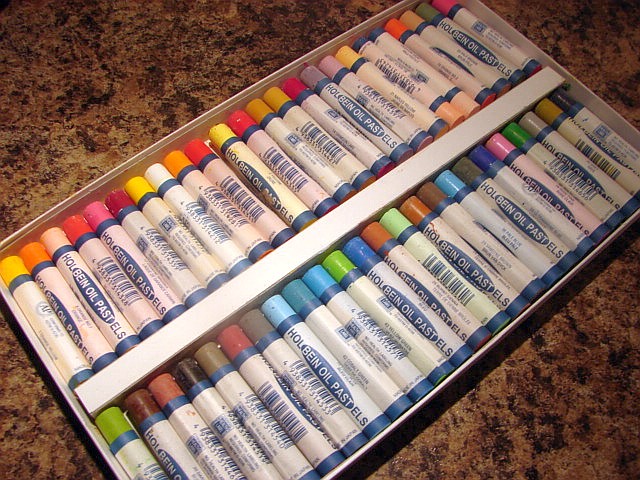This is an image of a large box of Holbein oil pastels lying open on a marble countertop. The countertop is characterized by a brown and black swirl, reminiscent of a type of granite often found in kitchens. The box is made of white cardboard and is currently without its lid. Inside, the pastels are arranged in two layers, separated by a white divider. Each layer seems to contain about 24 pastels, making a total of around 48. The pastels are presented in a wide range of colors including pink, red, yellow, white, orange, blue, green, brown, and black. They are not arranged by color; instead, they appear randomly placed with different hues next to one another, such as browns adjacent to pinks and greens. The pastels are lighter in color compared to regular crayons and are neatly lined up within the box, which rests entirety in the frame of the picture.